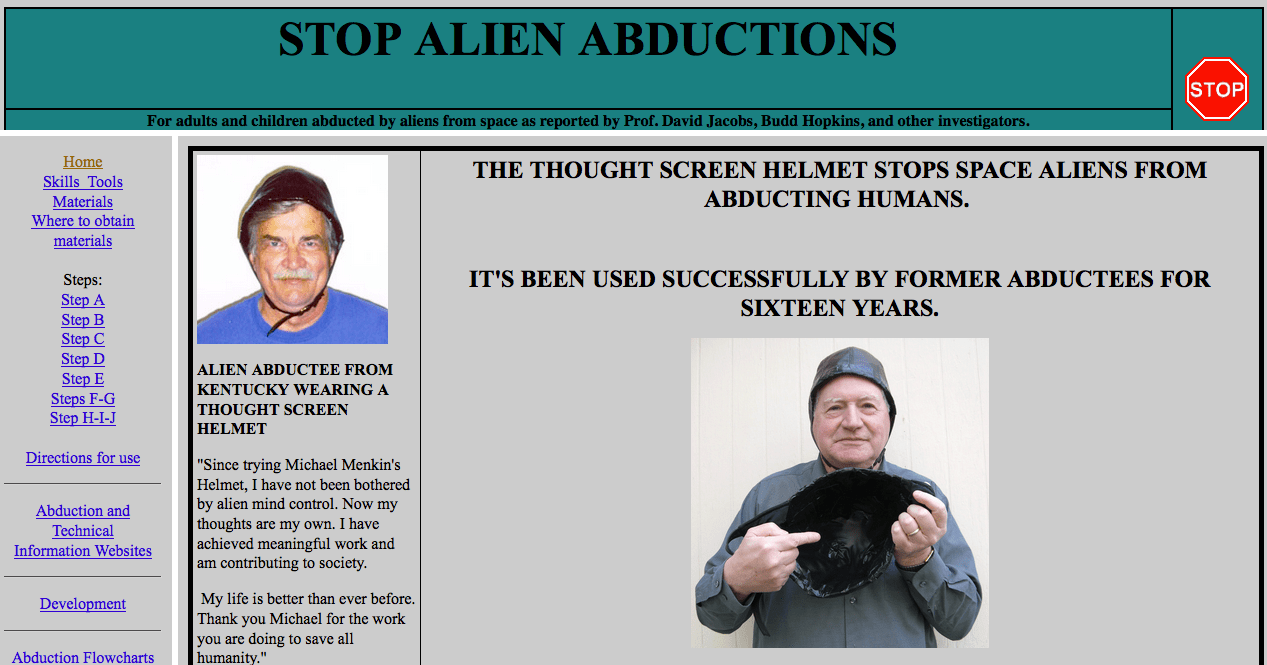The image depicts a computer screen showing a layered webpage focused on anti-alien abduction measures. The background page features a green backdrop with the text "Stop Alien Abductions" prominently displayed. The right-hand corner includes a partial view of a stop sign. Superimposed on this background is a large gray rectangle that centers the text "The Thought Screen Helmet Stops Space Aliens From Abducting Humans," followed by "It's been used successfully by former abductees for 16 years," all set against the light gray background.

Beneath this text is an image of an older white man holding a black object resembling the inside of a helmet. He is dressed in a gray hood and a gray long-sleeved shirt, also wearing a wedding ring on his left hand. Another image on the left side of the gray screen shows a different older man with a gray mustache, sporting a black chin-strap hat and a blue shirt with a white background.

The text accompanying this second image reads, "Alien Abductee from Kentucky Wearing a Thought Screen Helmet." Below is a testimonial about the effectiveness of the helmet, citing improvements in the man's life since using it. The far-left side of the gray screen contains navigation links in blueprints such as Home, Skills, Tools, Materials, Where to Obtain Materials, Directions for Use, and Development.